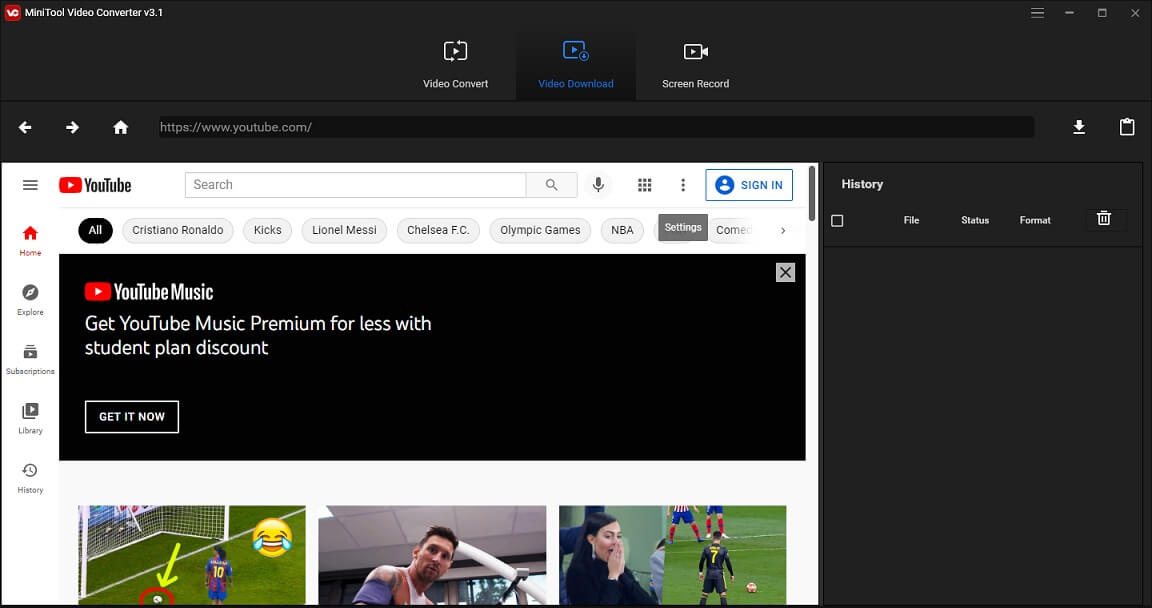The image is a screenshot of a computer screen displaying a black background, except for a prominent white rectangle on the bottom left corner. At the top of this white rectangle, three icons are visible: "Video Content," "Video Download," and "Screen Record," with the "Video Download" icon highlighted in blue, indicating it is selected. Above these icons, there are navigation buttons including an arrow pointing backward, an arrow pointing forward, and a home icon. 

A darker black rectangle appears to contain a URL, presumably indicating a web address typed into it. Inside the white rectangle, the word "YouTube" is positioned at the top left, accompanied by a search bar and a blue "Sign In" button on the right side. Multiple tabs for various selections are spread across the interface. Below these tabs, a wide black banner reads, "YouTube Music: Get YouTube Music Premium for less with Student Plan Discount. Get it now."

Beneath the banner, three partially visible images are evenly spaced out, though their lower portions are cut off. The mixture of navigational elements and promotional content showcases a typical browsing interface on YouTube’s website.